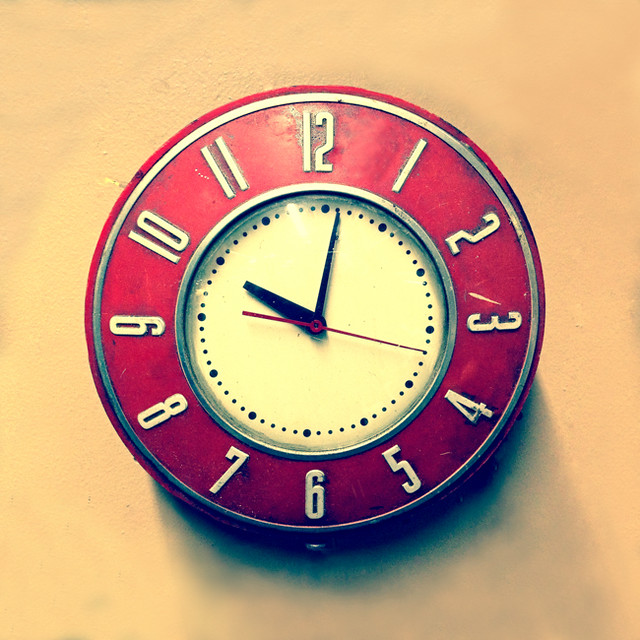The image depicts a vintage clock with a striking red frame, hanging on a cream-colored wall that has a slight yellow-orange tint, likely due to the photo's editing. The clock has a thick red border approximately 2-3 inches wide, and features large, white traditional numbers (12, 1, 2, 3, etc.) that are easily readable. Its face is adorned with black hour and minute hands, while the second hand stands out in red. The clock face also includes a series of dots, which appear to aid in telling the time: larger dots mark every five-minute interval, providing an additional level of clarity. The overall composition of the image is square, emphasizing the clock as the focal point against the subtly tinted backdrop.